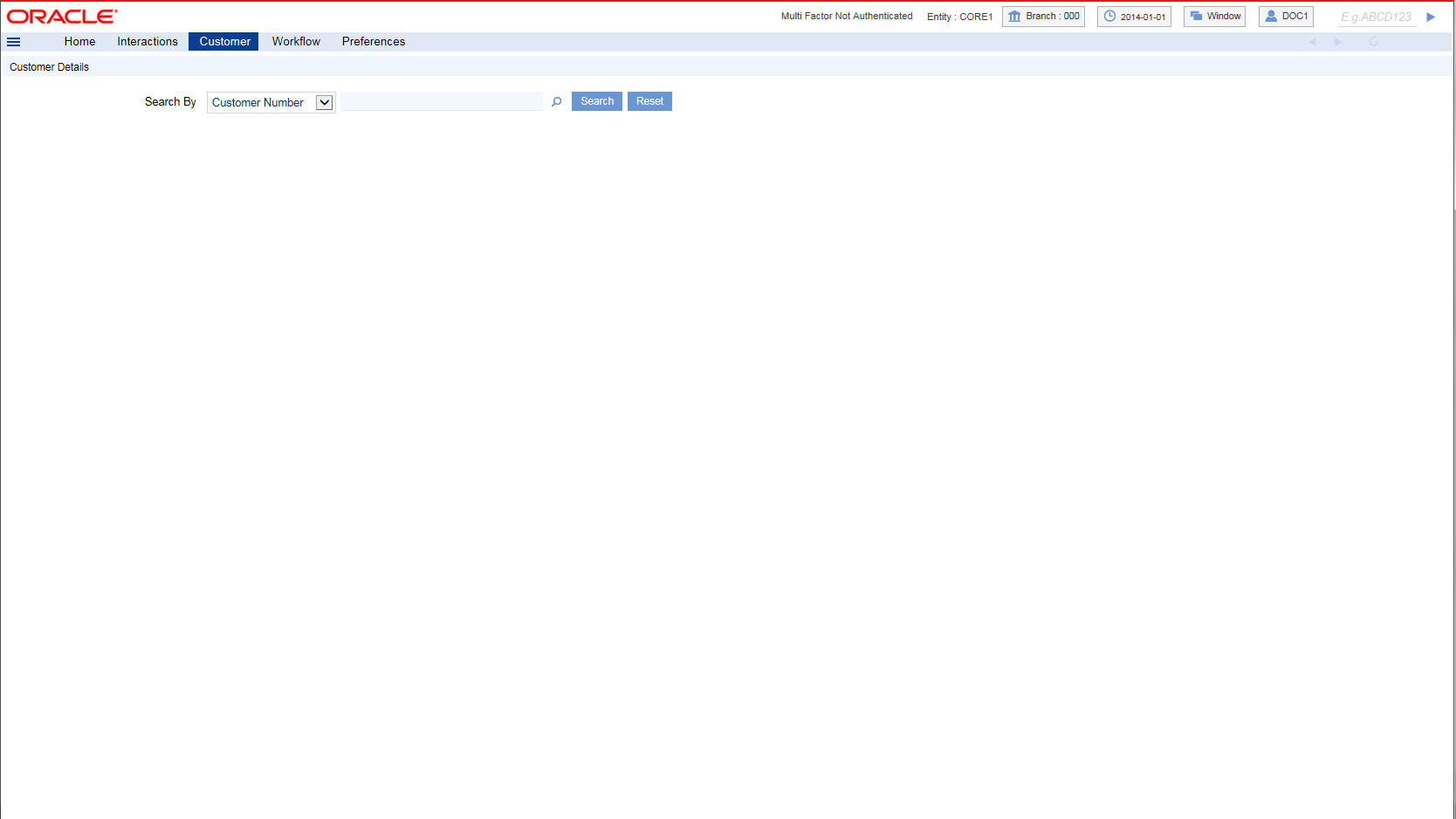A screenshot of the Oracle software interface displays prominently on a plain white background with minimal content. The top left corner features the recognizable red Oracle logo in a sleek, futuristic font. Across the top of the interface, several navigation tabs labeled "Home," "Interactions," "Customer," "Workflow," and "Preferences" are visible, suggesting various functional areas of the software. The user is currently on the "Customer" tab, which is mostly blank, indicating either an ongoing update or an absence of data.

Below the navigation tabs, there is a "Search By" button that enables users to search for information using customer number or other parameters. Additionally, in the top right corner, there are technical details related to Windows and branch settings, hinting at backend functionalities and potentially indicating this is an enterprise software used for managing business, workflow, and productivity. The overall design is utilitarian and not aimed at consumer interaction, reinforced by the significant empty space and the clean, unembellished layout.